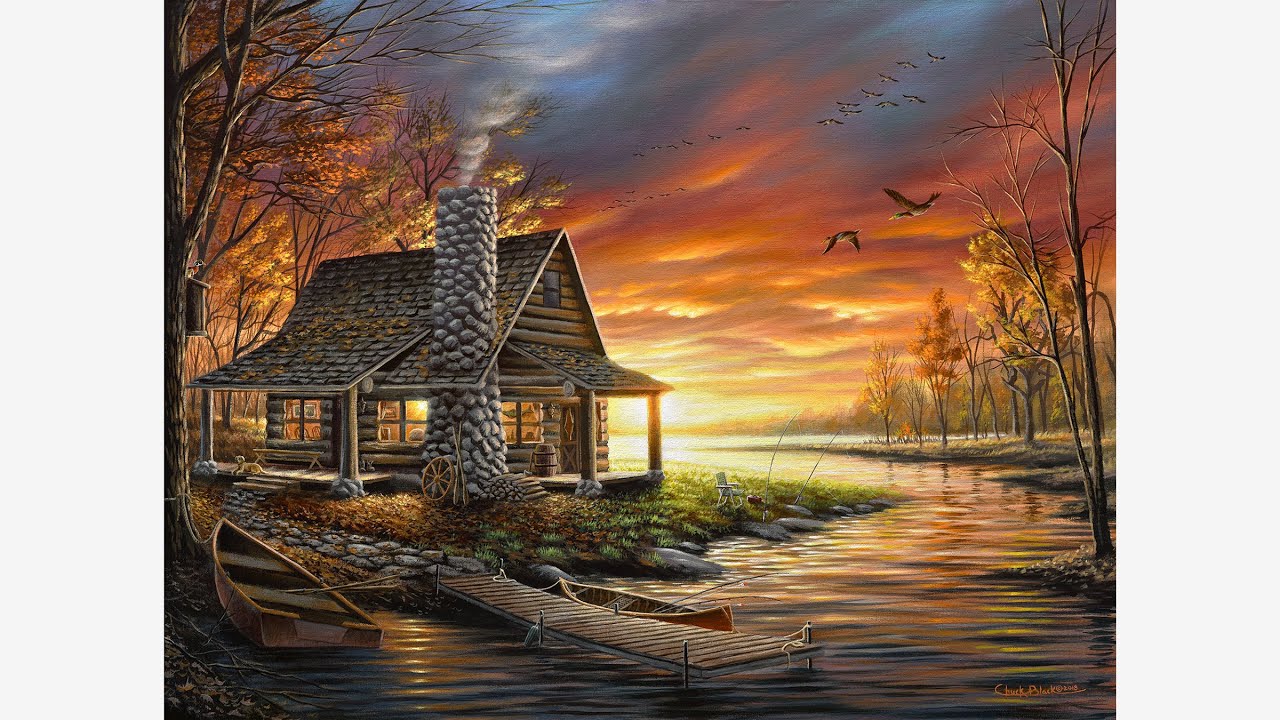The painting captures a serene lakeside scene at sunset. Dominating the left side of the image is a charming log cabin with a peaked, shingled roof and a wrap-around porch. A large stone chimney, emitting a thin trail of smoke, hints at the cozy warmth inside, which is dimly lit. The cabin’s dark wooden exterior is highlighted by the orange and yellow hues of the setting sun, which casts a warm, inviting glow across the landscape.

In the foreground, a stone path leads to a wooden dock that extends into the water, where a pair of canoes and a rowboat are moored, suggesting recent or upcoming adventures. The water, situated on the right side of the painting, reflects the vibrant sunset colors, showing ripples that add a sense of movement and life to the scene.

The backdrop features several sparsely-leaved trees, with some fully adorned with rich autumn colors and others bare, indicative of late fall. Enhancing the idyllic setting, two geese are captured in mid-flight against the orangey-red sky. Additionally, there is a solitary chair placed by the lake, inviting viewers to imagine sitting there, soaking in the tranquil beauty.

In the bottom right-hand corner, the artist’s signature, though difficult to decipher, is present in an orangish font, further emphasizing the warm tones of the artwork. The overall mood of the illustration is both picturesque and serene, evoking a sense of peace and longing to visit such a beautiful, undisturbed place.